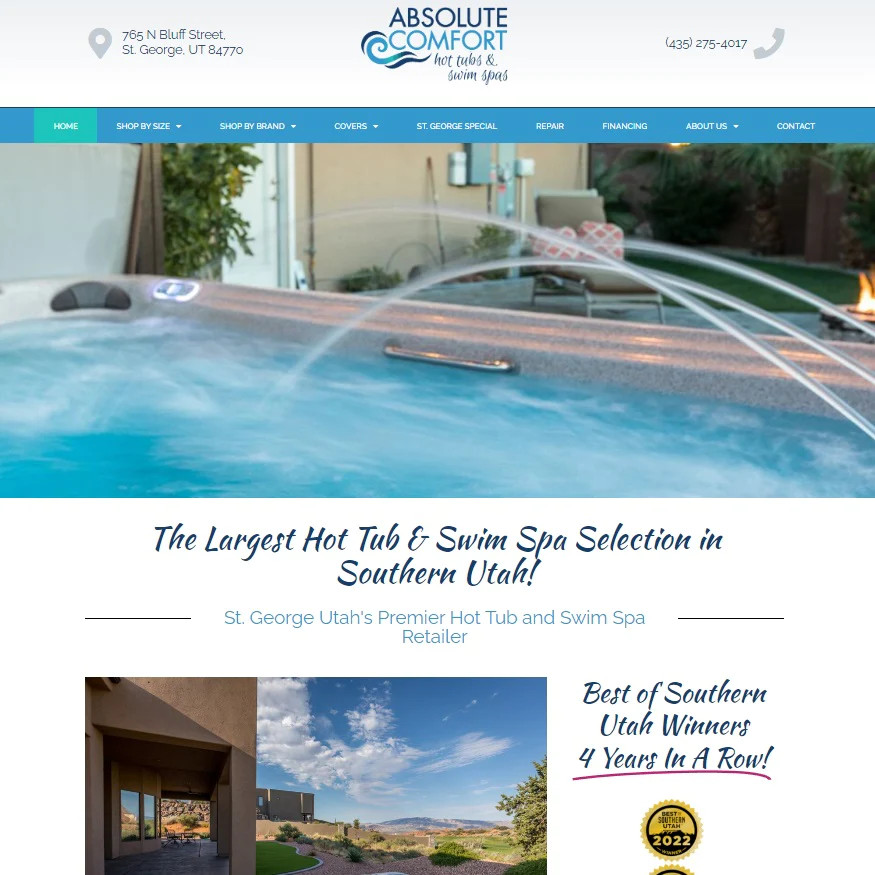The image depicts a screenshot of a website displayed on a computer, belonging to "Absolute Comfort," a business specializing in hot tubs and swim spas. The website's address is located at the top left corner, confirming its location in St. George, Utah. On the top right, there is a phone icon beside the business's contact number.

Below these details, a blue navigation bar stretches across the page, containing various clickable options. Some options are drop-down menus, while others redirect to different parts of the website. The current page is the home page, highlighted in a teal color. Other menu options include "Shop by Size," "Shop by Brand," "Covers," "St. George Special," "Repair," "Financing," "About Us," and "Contact."

In the main section of the website, there's a striking image of a luxurious hot tub with three streams of water gracefully arching on the right side. Accompanying the image, a text proudly states "The largest hot tub and swim spa selection in Southern Utah." Additionally, the business is noted for having received an award in 2022.